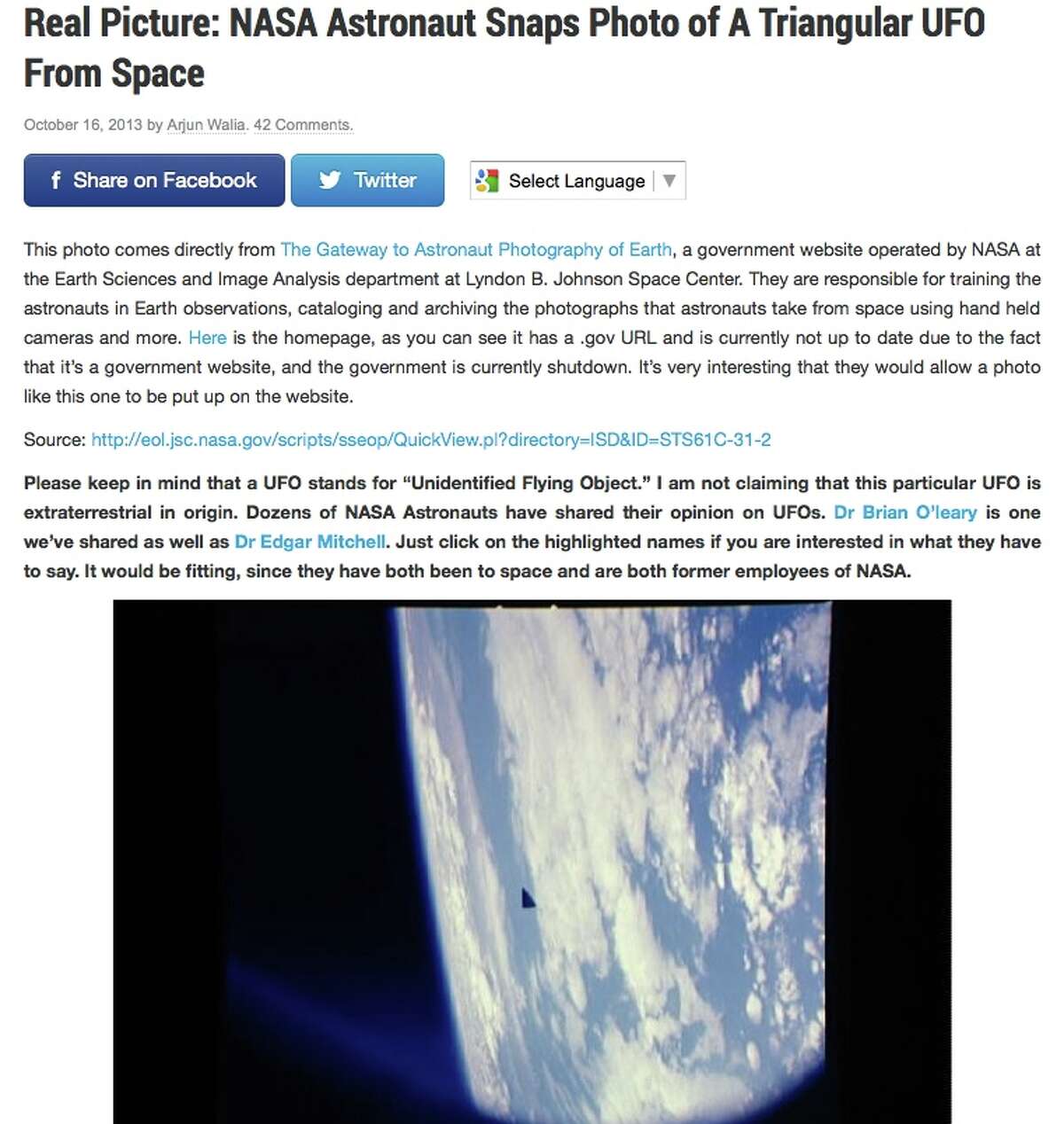A detailed caption for the described image could be:

---
Screenshot of an online article with a clean, white background. The article is roughly square-shaped and features a left-justified headline in large font that reads, "Real Picture: NASA Astronaut Snaps Photo of a Triangular UFO from Space." The word "Space" occupies its own line due to line break.

Below the headline, in small, light gray font, is the publication date "October 16, 2013" followed by the author’s name, "Arjun Walia." Both the name and the "42 comments" indicator next to it are faintly underlined, suggesting they are clickable for further interaction.

Underneath the author’s name, three horizontally-aligned rectangular buttons with rounded corners are visible. The first, a dark blue button featuring the Facebook "F" logo and the text, "Share on Facebook." The second, a lighter blue rectangle containing the Twitter bird icon with the word "Twitter." The third is a smaller dropdown field with a multicolored square on the left, labeled "Select Language," and includes a downward arrow indicating a menu.

The article's content starts beneath these buttons, with justification on both sides. The first paragraph spans six lines, stating that "This photo comes directly from The Gateway to Astronaut Photography of Earth," with the clickable phrase in light blue font linking to NASA's website. A blank space follows this paragraph, succeeded by a bolded four-line paragraph emphasizing, "Please keep in mind that a UFO stands for 'Unidentified Flying Object.' I am not claiming that this particular UFO is extraterrestrial in origin," with names like Dr. Brian O'Leary and Dr. Edgar Mitchell in clickable blue font, indicating references to valid sources or articles.

Following the text is the actual photograph discussed in the article. The image itself is landscape-oriented and slightly wider than its height. The majority of the photograph is black, with a vertical section of sky and clouds positioned nearly at the center, creating a 40% vertical stripe. Within this sky section, almost dead-center, appears a small black triangular object identified as the UFO.
---